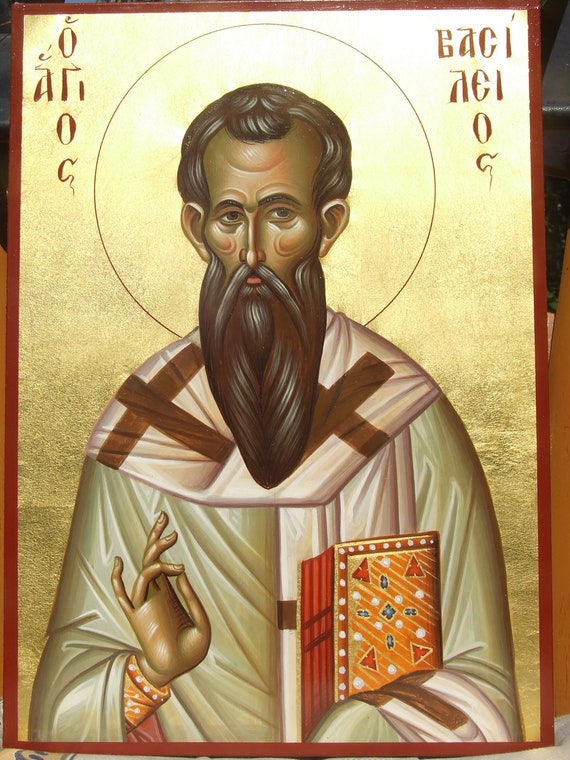This is an illustration of a religious figure, possibly a priest or Saint Basil, depicted in a portrait orientation with detailed Byzantine iconography. The man, with short black hair, a long black beard, and a thin mustache, is dressed in ornate white robes featuring large red crosses on the sleeves and a matching draped scarf over his shoulders. His right hand is held up with the thumb touching the ring finger, forming a gesture that’s almost an 'okay' sign, while his left arm cradles an ornate, orange-covered book adorned with symbols and geometric patterns. His face exhibits artistic swirls and a somewhat unrealistic, impressionistic quality. Surrounding his head is a golden halo, indicative of his sanctity, highlighted against a rich gold leaf background. The image is framed with a brown border, and there is indecipherable, non-Roman script in the upper corners that suggest foreign origin or ancient religious text. The overall color scheme includes brown, orange, white, red, and hints of pink, contributing to the divine and sacred ambiance of the illustration.